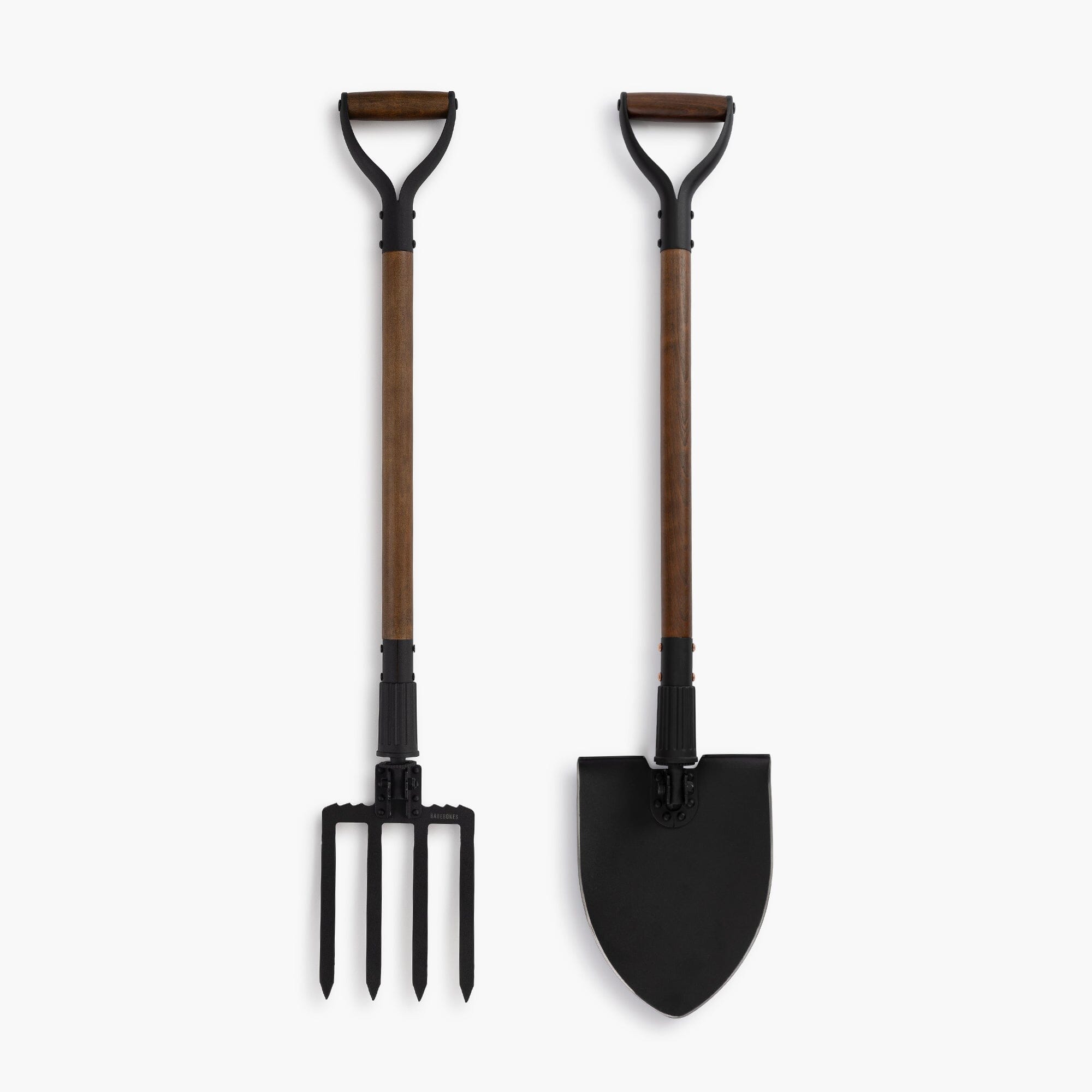This detailed photograph showcases two gardening tools against a faint light gray, almost white background. The image is square in shape, approximately six inches by six inches. Centrally aligned, the tools are arranged vertically with handles at the top and implements at the bottom. On the left side is a four-tined pitchfork, and on the right, a broad spade-shaped shovel. Both tools share similar design characteristics: black metal handles with dark mahogany brown wraps, wooden shafts in a deep brown hue, and dark metal ends. The pitchfork is slightly shorter than the shovel, with both tools measuring around four inches in height. Notably, the necks of these tools feature joints indicating they can be collapsed or extended, suggesting a portable design possibly influenced by military or multi-functional utility gear.